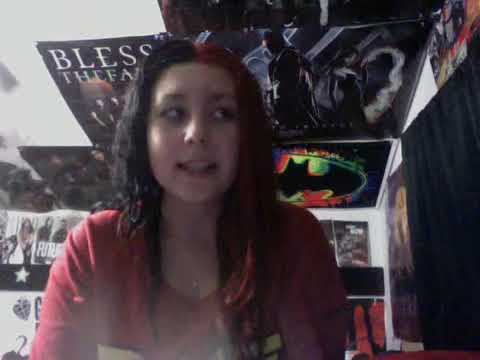The image is a small, somewhat blurry photograph of a young Caucasian woman centered in the frame from mid-chest up. She has long, wavy hair that is black on one side and dyed red on the other, parted in the center. Her face is towards the camera, but her eyes are looking to her right. Her mouth is open slightly, as if she is speaking, revealing her teeth. She is wearing a red crew-neck T-shirt, though the sleeves are not visible as the photo cuts off just below her chest. There is indistinct yellow lettering on her shirt. Around her neck is a necklace. The background depicts a room with mostly white walls and a ceiling largely covered with posters, adding a busy and cluttered feel. Notable posters include one with the partial text "bless the..." above her head and a visible Batman poster near her right shoulder. The rest of the posters are blurred and difficult to identify, contributing to the overall slightly grainy and older appearance of the photograph.